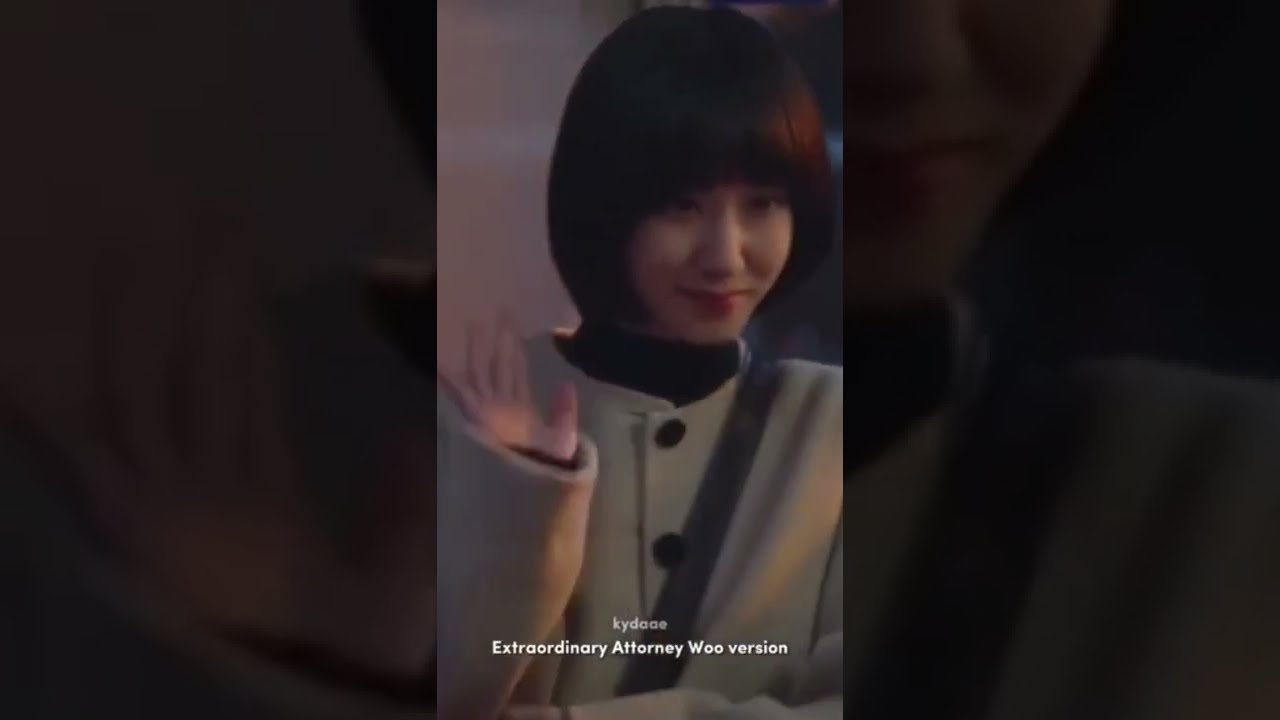The image features a vertical cell phone picture of an Asian woman centered against a darkened and zoomed-in background that is actually a faded, extreme close-up of the same woman. She has a bowl cut with bangs and is smiling with her mouth closed. She is dressed in a cream-colored, heavy wool coat with black buttons and is wearing a black turtleneck underneath. The woman also has a purse strap visible on her left shoulder. She appears to be waving with her right hand. The image is a close-up, cropped at her shoulders, and she is looking slightly downward. Near the bottom, white text reads "Extraordinary Attorney Woo Version," with a partially obscured word above that could be "VIADOAE." The background on the left and right is dark and underexposed, creating a focus on the well-lit subject in the center.